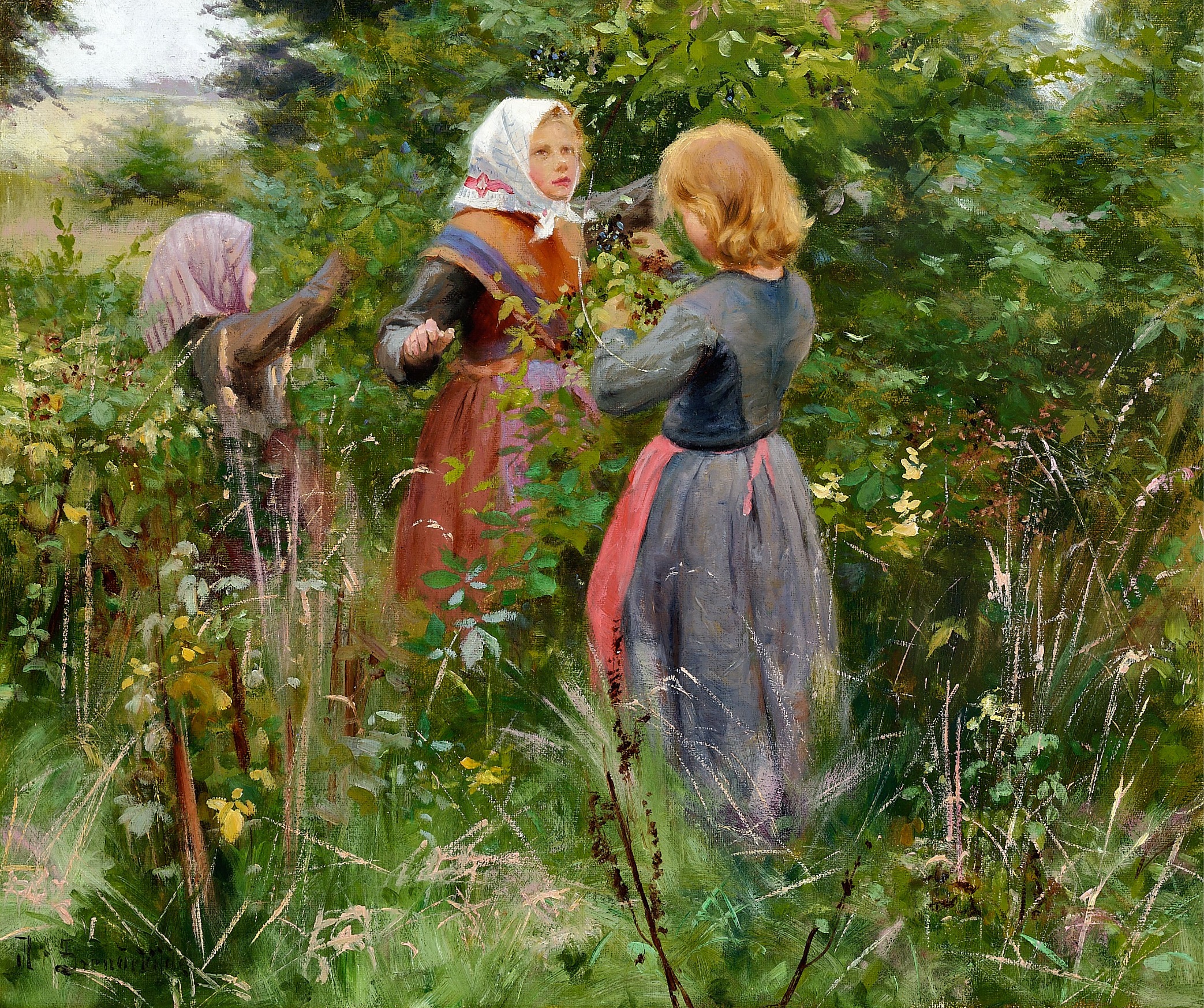In this highly realistic painting or photograph, we see three young girls amidst a lush, rural landscape, possibly picking berries. The girls are dressed in long, working dresses that reach their hands and feet, standing among tall grasses, flowers, and berry-laden shrubs. The girl in the middle, wearing a brownish-orange dress and a white scarf with red on her head, gazes thoughtfully up and to the right, as if lost in thought or observing something in the sky. To her left, another girl in a gray dress with a pinkish apron and a purple scarf appears to be reaching into the bushes, possibly picking berries. The girl to the right, whose back is turned to us, wears a gray dress with a hint of red on the front. She is focused on the task in front of her, perhaps gathering berries from the bush. The scene is set within dense foliage with some flowers and a distant field visible in the upper left corner, contrasted against a lighter sky, creating a picturesque and serene rural setting.